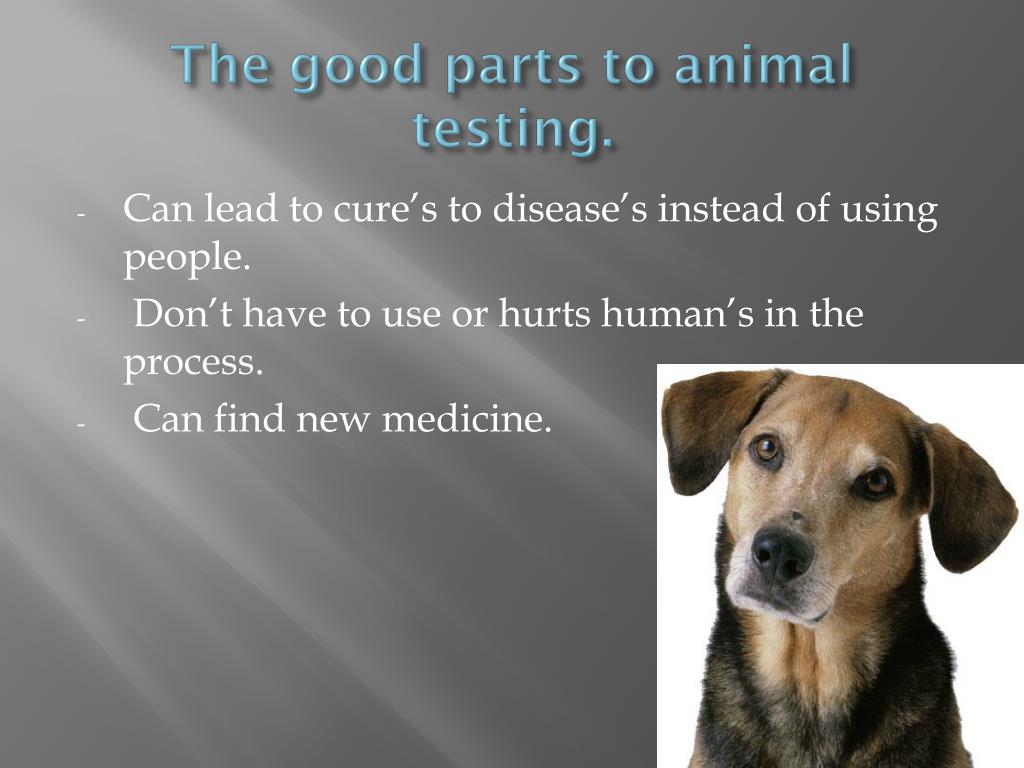This image appears to be a slide from a PowerPoint presentation. The background is predominantly dark gray with a gradient of white streaks emanating from the top left corner, giving the impression of light rays or illumination. At the top, centered in blue text, the title reads, "The good parts to animal testing." Below this, there are three left-aligned bullet points in white text. The first bullet point states, "Can lead to cures to diseases instead of using people." The second point reads, "Don't have to use or hurt humans in the process." The third and final bullet says, "Can find new medicine." Each point starts with a capital letter and ends with a period. In the lower right-hand corner, there is a white rectangular box containing an image of a dog. The dog, a mix of light brown and darker brown with patches of black, is looking directly at the camera with its head tilted to the right, evoking a sympathetic expression. Its face features a lighter brown shade with a touch of white around the muzzle, a black nose, and floppy, dark brown ears. The neck area transitions from lighter brown to darker shades.